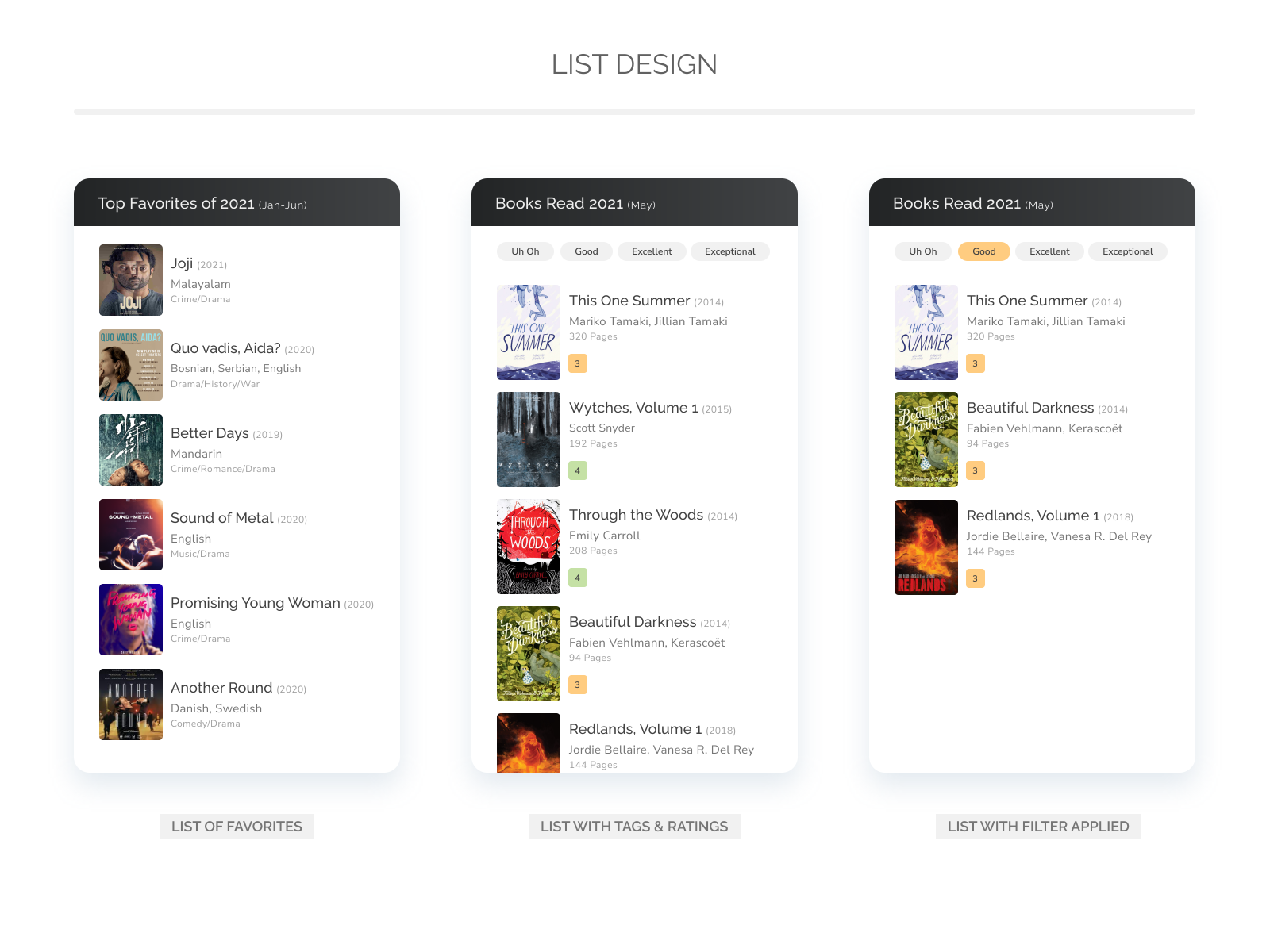**Detailed Caption:**

We are viewing a screenshot of a web page titled "List Design". The page is organized into three vertical columns, each resembling the dimensions of a cell phone screen, and displayed horizontally across the monitor.

Starting from the left column, the heading reads, "Top Favorites of 2021: January through June". This section contains a list of items:
- Joji
- Kuo, Vadis, Ida
- Better Days
- Sound of Metal
- Promising Young Woman
- Another Round

The center column is labeled "Books Read in 2021: May" and lists several books along with their ratings. The books listed are:
- This One Summer
- Witches, Volume 1
- Through the Woods
- Beautiful Darkness
- Redlands, Volume 1 (the rating for Redlands is cut off at the bottom of the page)

The ratings are presented via a bar at the top indicating levels such as "U-H-O-H", "Good", "Excellent", and "Exceptional". None of the books reach the top rating bar. Individual book ratings are as follows:
- This One Summer: 3
- Witches, Volume 1: 4
- Through the Woods: 4
- Beautiful Darkness: 3

The right column, also under the section "Books Read in 2021", duplicates some of the books listed and shows standardized ratings marked as "Good". The books displayed are:
- This One Summer
- Beautiful Darkness
- Redlands, Volume 1

All three listed books in this section are rated as "Good" with a rating of 3 each. The bottom of the center image features a button labeled "List with Tags and Ratings", while the bottom of the right image has a button labeled "List with Filter Applied". At the very bottom, there's a button titled "List of Favorites".

The overall background of the web page is a light grey or off-white, with a grey bar running across the top of the page. The central heading, "List Design", is prominently displayed at the top.